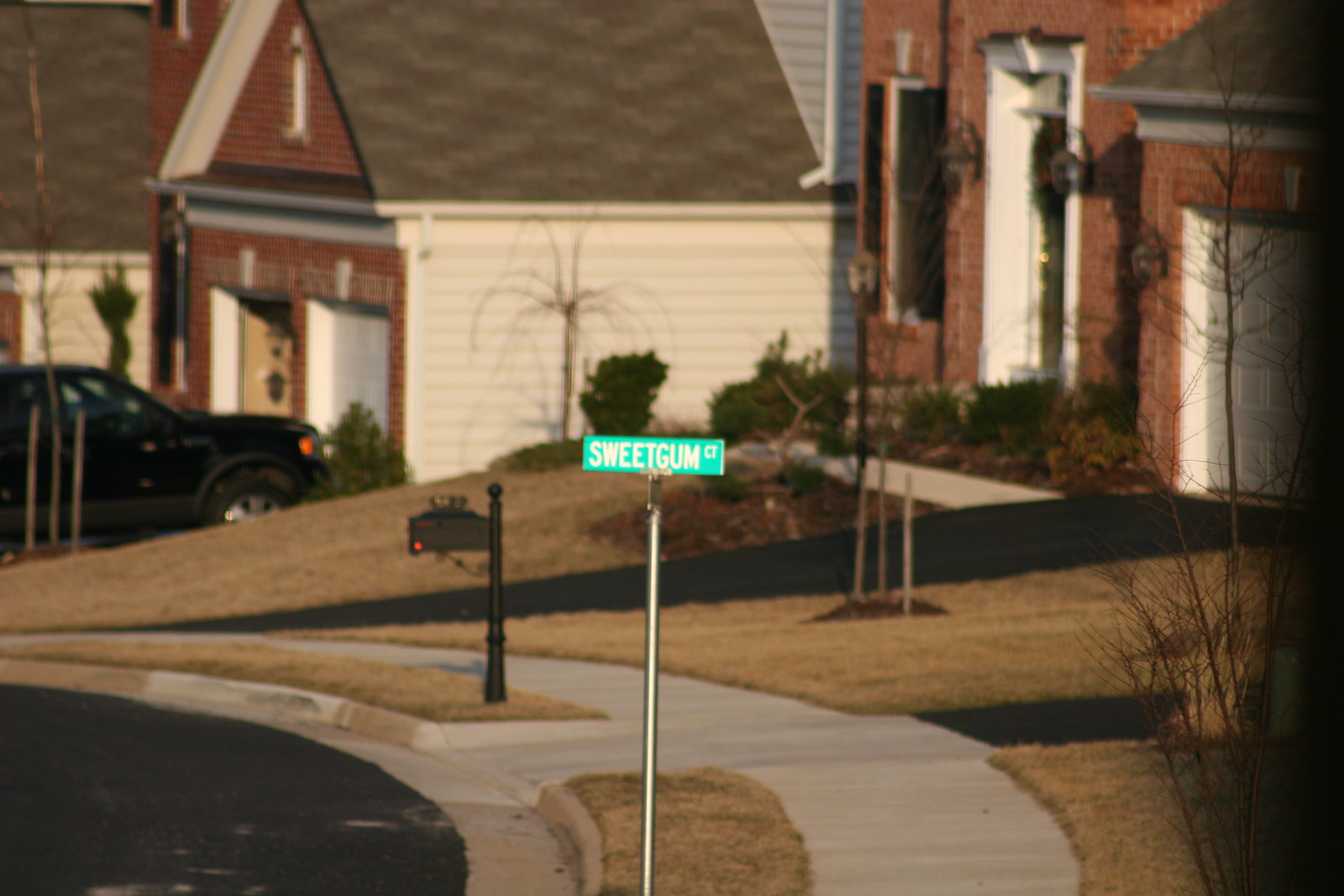The image captures a serene residential neighborhood scene. Central to the photo is a green street sign reading "Sweet Gum Court," prominently mounted on a metal pole extending down through the bottom center of the image. To the right of the sign is a well-maintained sidewalk. Directly behind the sign, a blacktop driveway slopes upward, featuring a black mailbox marked with a small red dot at the lower left corner. This driveway leads to a charming brick house with a pristine white garage door. Adjacent to the driveway is another sidewalk that ascends a couple of steps to the house's white front door. Beside this house is another brick residence with a garage complemented by white siding, and in its driveway, a black vehicle is parked. The entire scene exudes a sense of suburban tranquility and meticulous upkeep.